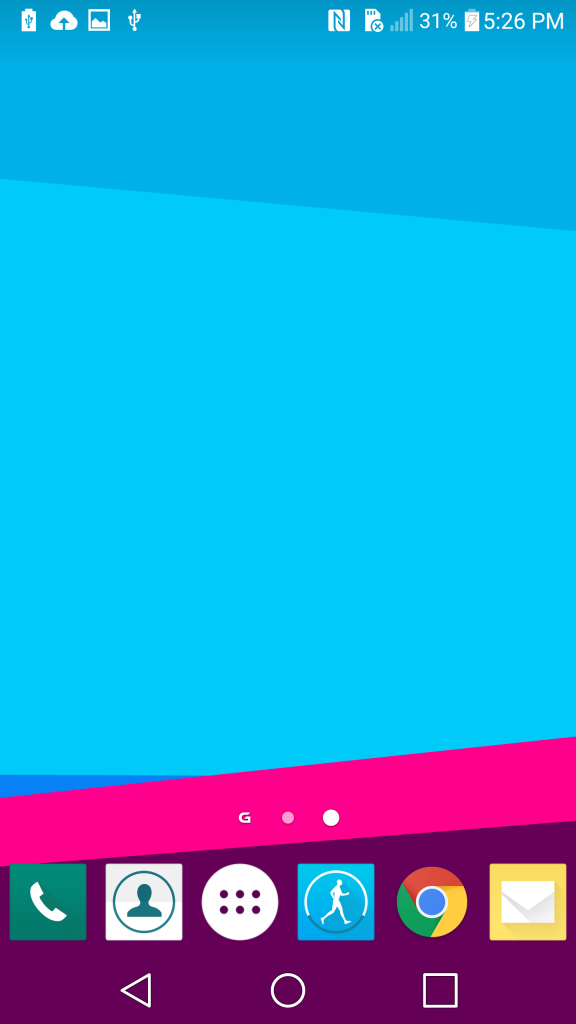The image depicts a complex interface with a richly colored background and numerous icons and symbols. The background transitions from dark blue at the top to mid-blue in the center, baby blue beyond that, a small band of darker blue, and finally into hot pink at the bottom. 

At the bottom bezel, a dark green square displays a white silhouette of a phone, adjacent to a white square with a black circle that features a silhouette of a person in dark black or dark blue. Nearby, a circular icon contains six smaller circles within it, set against a maroon-purple background, representing an app selection feature.

At the top, two ellipses, with the second ellipse highlighted and the first in grey, are followed by a white "G." A cyan-blue square nearby encompasses a cyan-blue circle with a partly white border and a black lower portion, featuring a silhouette of a walking person.

The familiar Google Chrome logo is present, divided into thirds of red, green, and yellow sectors converging on a central blue circle with a white border. Additionally, a gold-yellow square displays a white envelope with a dark gray shadow on its right side.

In the upper section, a battery icon shows it's charging via USB, accompanied by a cloud with a black up-arrow. Other symbols include a square with white mountains, another USB indicator, a pair of white "N" shapes, an SD card icon, and a white circle with a black "X" and a border, along with a cell signal icon with zero bars, indicating potential SIM card issues.

A percentage readout of 31% is next to a battery symbol nearly full, showing it's charging from about 33% to full capacity, marked by a central lightning bolt. Finally, the time "5:26 PM" is displayed on the right-hand side.